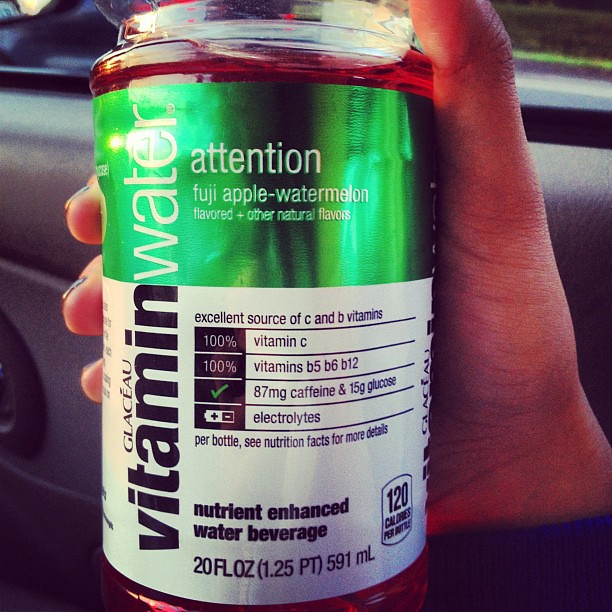This photograph captures a close-up of a hand, possibly a woman's, holding a plastic bottle of Glaceau Vitamin Water in a car setting. The skin tone appears to be brown or red, suggesting a non-Caucasian ethnicity. The sports drink bottle features a distinctive two-tone label, with the top portion in shiny foil green and the bottom portion in white. The text on the label includes "Vitamin Water Attention," specifying the Fuji Apple Watermelon flavor with other natural flavors. The green part of the label displays white text, while the white part has black text detailing its nutrient contents. The drink is described as a nutrient-enhanced water beverage providing 120 calories per 20 fluid ounces (591 milliliters or 1.25 pints) per bottle. The label highlights an excellent source of vitamin C and B vitamins (B5, B6, B12), alongside 87 milligrams of caffeine and 15 grams of glucose. Furthermore, it contains electrolytes, represented by a battery icon, and features a table that details the percentages of daily vitamin values. The label includes a note to see the nutritional facts on the back for more detailed information.